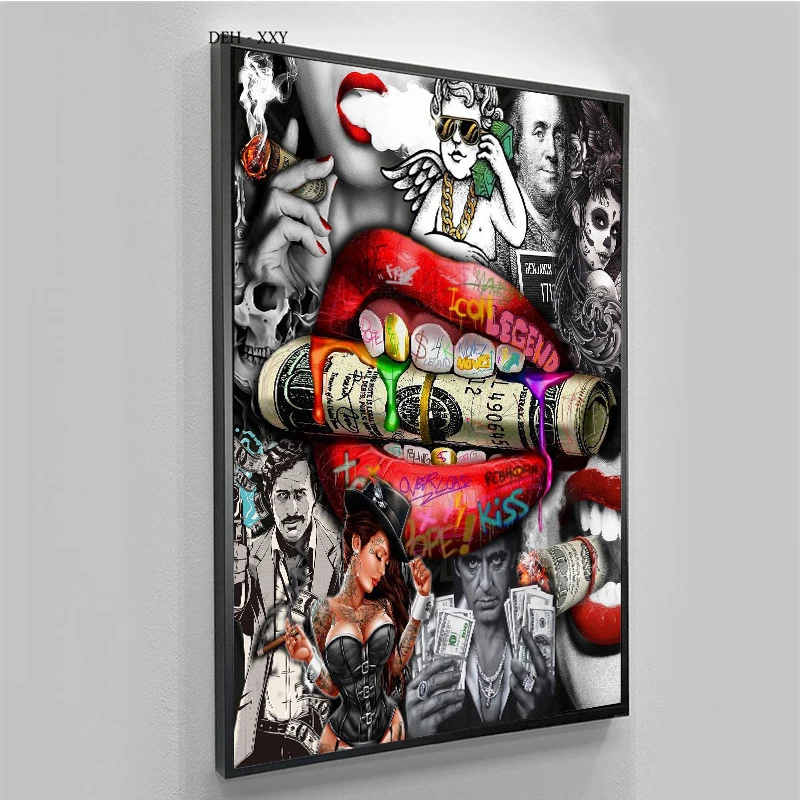This image features a vibrant and eclectic painting prominently displayed on a wall, possibly within a gallery or private collection. The painting is surrounded by a sleek black frame and contains a dense collage of pop culture elements and symbolic imagery, emphasizing themes of wealth and materialism.

At the heart of the artwork is a striking set of red lips, evocative of the Rolling Stones logo, but with a twist: one of the teeth is gold, and the remaining teeth display various numbers and writings in a graffiti style. These lips are assertively biting down on a rolled-up wad of hundred-dollar bills, with vivid streaks of red, orange, green, and purple paint cascading down the side of the money.

Encircling the central lips are a multitude of intriguing and disparate images. Among them is a depiction of Al Pacino, perhaps in his iconic role from "Scarface" or "The Godfather," gripping fistfuls of cash. The painting also includes Benjamin Franklin's portrait, a gold-chained, sunglasses-wearing Cupid-like angel holding a stack of green money as a telephone, and an airbrushed skull contributing to the dark, edgy aesthetic.

On the periphery, we see another set of lips, with a woman's face partly visible, exhaling smoke from a cigar composed of rolled-up bills, enhancing the opulent theme. Additionally, there is a vaudeville dancer clad in a bustier and fedora, and a figure reminiscent of El Chapo.

The top corner of the photograph showcasing the painting features a watermark reading "Dell XXY." The piece as a whole pulsates with a vivid color palette dominated by reds, greens, and other bright hues, encapsulating a dynamic, garish, and highly materialistic visual narrative.